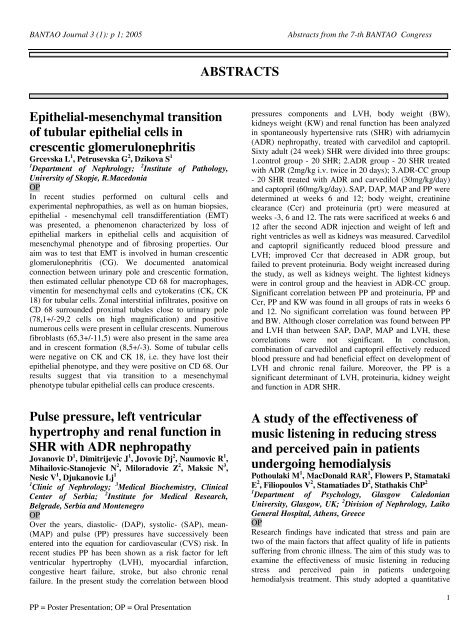This black and white image depicts a page from the Bantao Journal, specifically from the year 2005, Volume 3, Issue 1, Page 1. The page is titled "Abstracts from the 7th Bantao Congress," with the word "Abstracts" prominently positioned between two gray bands. The page showcases three scientific abstracts. The first abstract, "Epithelial Mesenchymal Transition of Tubular Epithelial Cells in Crescentic Glomerulonephritis," authored by L. Grzeszewska, G. Petruszewska, and S. Zipova from the Department of Nephrology, Institute of Pathology, University of Skopje, Macedonia. The second abstract, "Pulse Pressure, Left Ventricular Hypertrophy, and Renal Function in SHR with ADR Nephropathy," is credited to D. Jovanovich and colleagues from the Clinic of Nephrology, Medical Biochemistry, Clinical Center of Serbia, Institute for Medical Research, Belgrade, Serbia and Montenegro. The third abstract, "A Study of the Effectiveness of Music Listening in Reducing Stress and Perceived Pain in Patients Undergoing Hemodialysis," is authored by M. Potulati, R. A. R. McDonald, and others from the Department of Psychology, Glasgow Caledonia University, University of Glasgow, UK, and the Division of Nephrology, Lyco General Hospital, Athens, Greece. The small textual details, though barely readable, contribute to the formal and structured layout typical of academic journal pages.